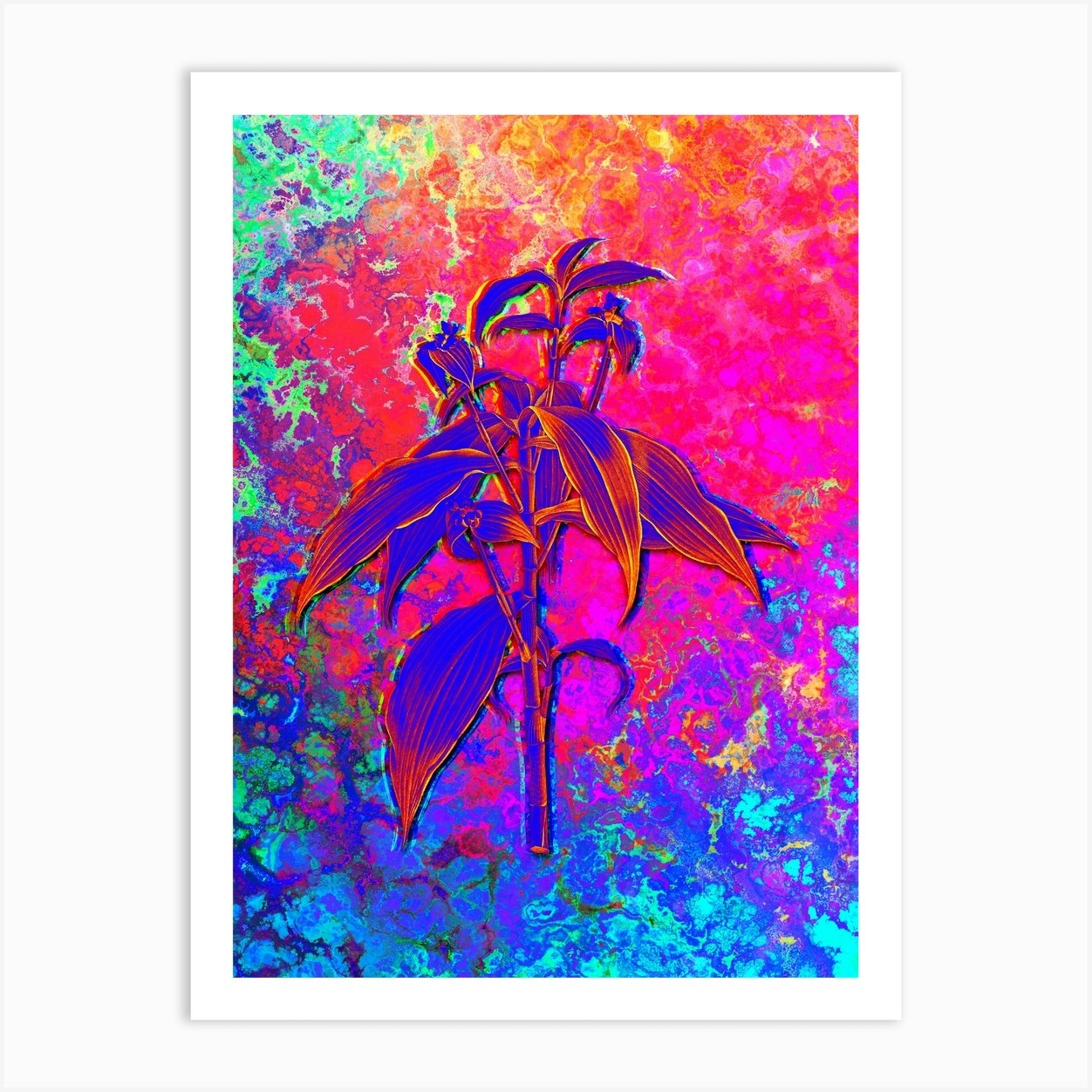This abstract art image, displayed on a white wall, features a vibrant, color-mottled background surrounded by a subtly contrasting white frame. The top left of the artwork is painted green blended with purple, transitioning to an orange area with crimson hues, further blending into shades of pink and orange. The bottom right is dominated by blues. At the center of this chromatic explosion, a visually compelling plant—possibly resembling a bamboo or corn stalk—bursts forth. The plant's stem displays an array of purple and orange, while its leaves and associated elements mix in blue, yellow, green, and purple. The piece exhibits a unique visual texture as if developed through a specialized photographic technique.